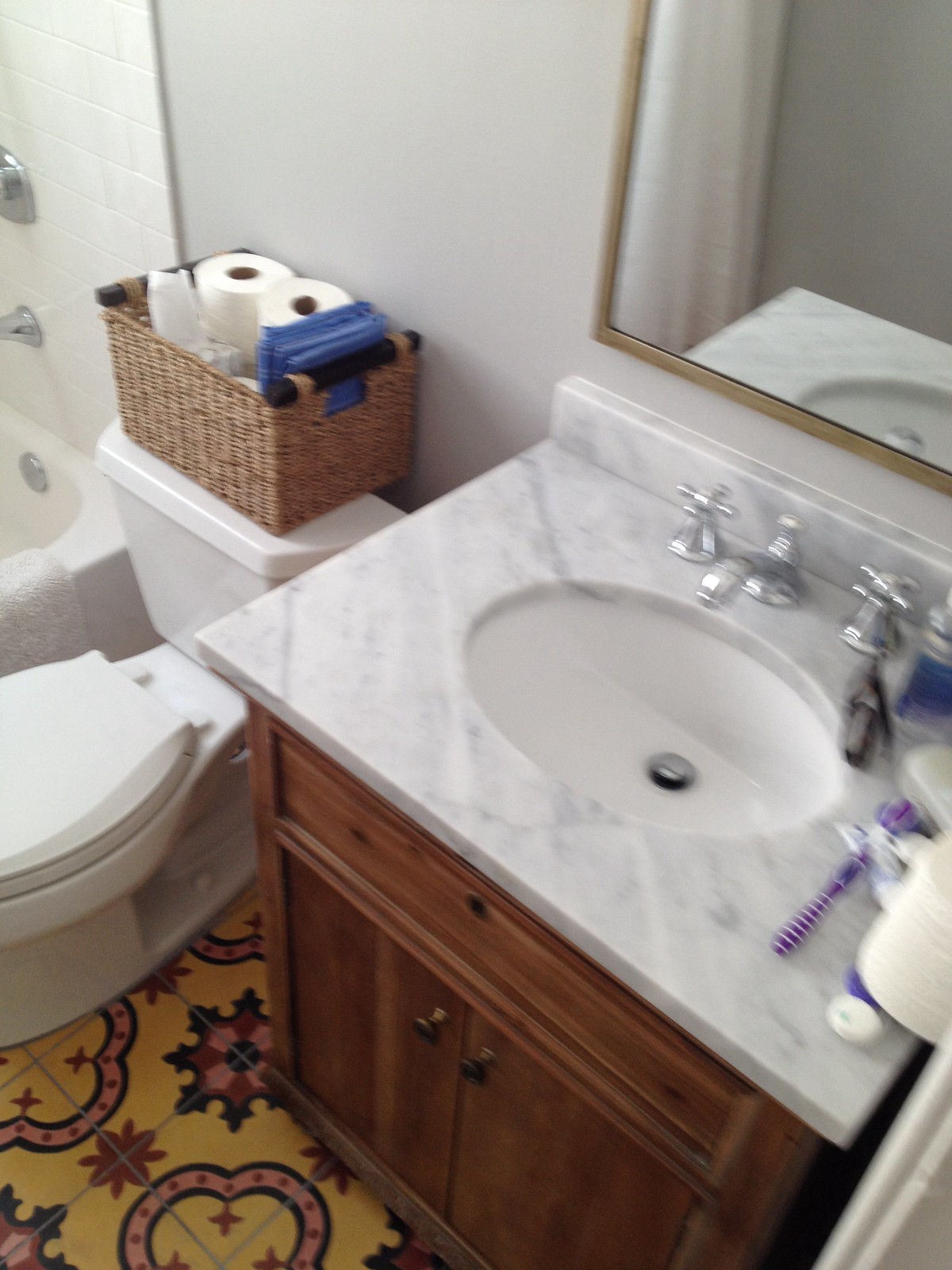This photograph captures a detailed view of a bathroom, showcasing an assortment of design elements and fixtures. The floor is the highlight with a striking and intricate pattern; it features a yellow background adorned with artistic designs. Each tile is unique, depicting vibrant images: some tiles feature a red star in the middle, while others showcase a large black star with a red circle at its core surrounded by yellow dots at the top, left, right, and bottom, encased by a black circle.

Central to the image is a standard white toilet. Atop its tank sits a brown rectangular basket that holds several items, including a roll of toilet paper and what appears to be a blue rag on its right side. To the left of the toilet, a small section of the bathtub is visible, including the faucet and the drain stopper mechanism.

On the right side of the photograph, the bathroom sink is nearly fully visible. The sink has an elegant oval shape and a luxurious gray and white marble-like design. A purple toothbrush resides on the sink, adding a splash of color. The silver knobs of the sink enhance its sophisticated appearance. Above the sink, a mirror is partially visible, reflecting light and expanding the visual space of the room. Below the sink, the cabinetry is a warm brown, creating a cohesive look with other wooden elements in the bathroom.

This carefully orchestrated arrangement of colors, patterns, and fixtures comes together to create a bathroom that combines functionality with stylish elements.